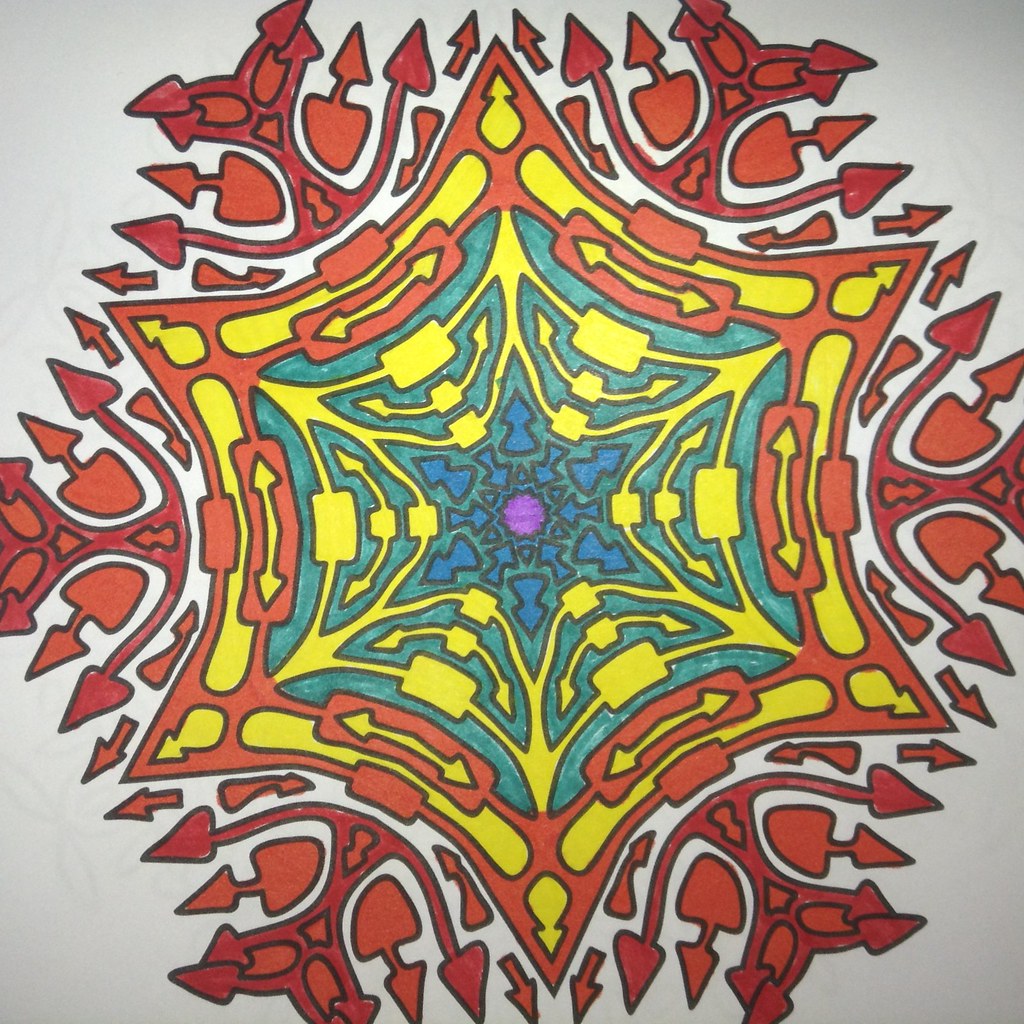The image is a vivid, intricate illustration set against a white background. At the very center, it features a deep purple core. Surrounding this core are blue arrows pointing outward, which transition into a larger blue star shape. This star radiates into an expansive yellow pattern enveloping it, which is then bordered by another shade of blue. Beyond this, a complex red pattern encircles the entire composition. 

Purple arrows, encased in rectangles, extend outward to the left and right, juxtaposing with inner yellow segments. The red pattern, composed of arrow-like shapes, diversifies in orientation, spreading left, right, and upward. The entire structure has a fractal-like quality, with its vibrant colors and geometric shapes propagating from the center towards the edges, creating a dynamic and eye-catching visual flow.